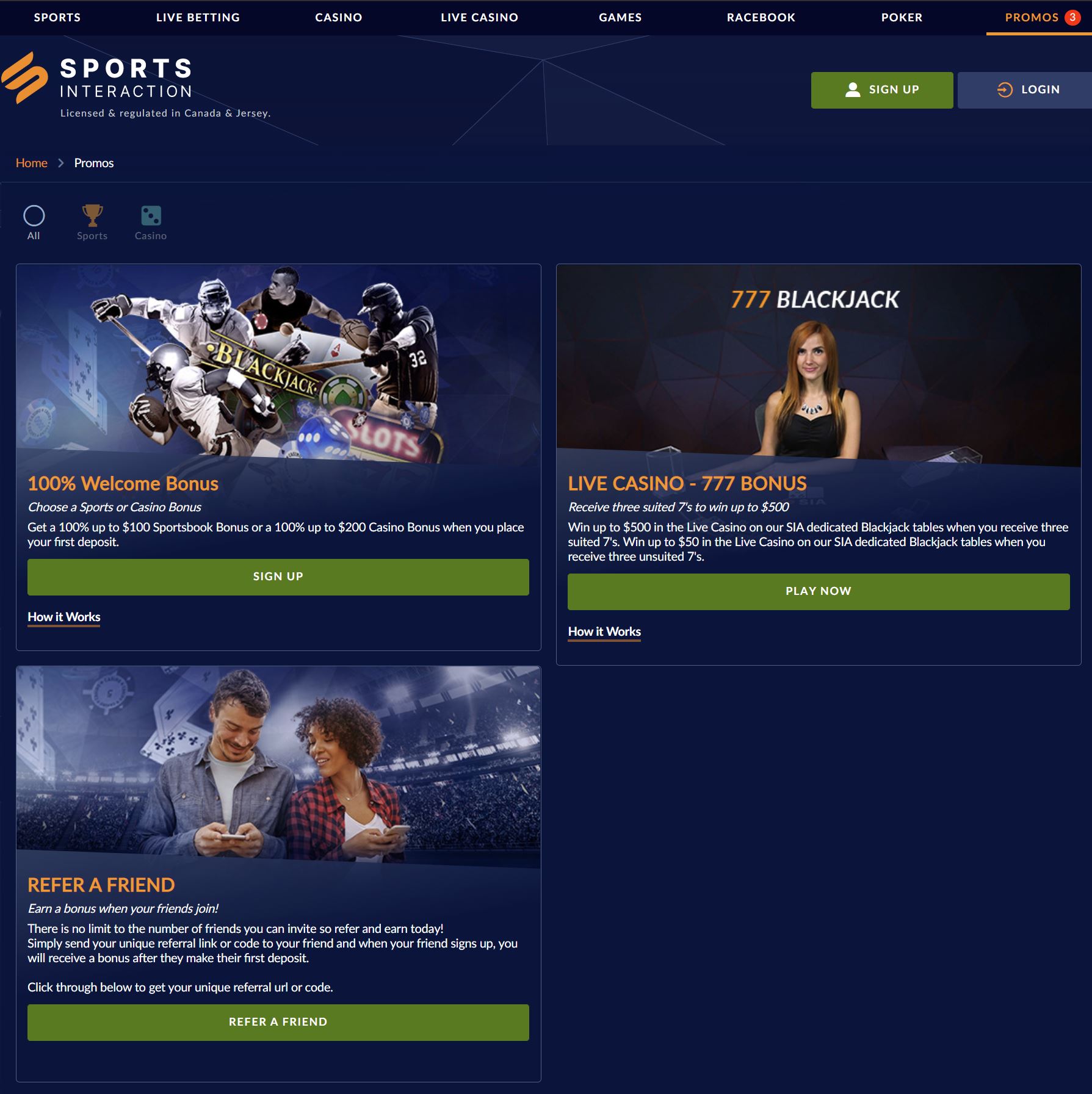This image depicts a screen capture of a predominantly navy and white website, likely related to online betting or gaming. At the top of the website, the menu options include "Sports, Live Betting, Casino, Live Casino, Games, Racebook, Poker, and Promos." The "Promos" tab is highlighted in orange with a small orange circle indicating the number "3." Below the menu, the website is branded with "Sports Interaction," and notes that it is "licensed and regulated in Canada and looks like Jersey." To the right, there are two prominent buttons: a green and white "Sign Up" button, and a navy, white, and orange "Log In" button. Additionally, there are options labelled "Home" and "Preferences."

Further, the site features three icons with different themes:
1. "All" – marked by a white circle.
2. "Sports" – symbolized by an orange trophy.
3. "Casino" – indicated by light blue dice.

Moving down the page, three separate promotional images offer various deals:
1. The first image promises a "100% Welcome Bonus." Users can choose between a sports bonus (100% up to $100) or a casino bonus (100% up to $200) upon their first deposit. A green "Sign Up" button with white text accompanies this offer, along with a straightforward "How it works" callout.

2. The second image features a redheaded woman in a black tank top and necklace, set against a black background. Above her head, the text "777 Blackjack" is highlighted in white and orange. The promotion offers a potential win of up to $500 in the live casino, specifically in a blackjack jackpot. This section also includes a green "Play Now" button with white font and another "How it works" note.

3. The third image depicts a couple – a woman in a plaid and white shirt with curly black hair and a man in a blue and white shirt. Both are holding cell phones. Behind the man’s shoulder, some playing cards are visible, and by the woman, there appears to be a stadium setting. The text reads "Refer a Friend," encouraging users to earn a bonus when their friends join. Below this, a paragraph explains the process and instructs users to "click through below to get your unique referral URL code." A green button labeled "Refer a friend" is also included.

Overall, this screen capture showcases a well-organized website with various sections for betting and casino games, along with enticing promotional offers.